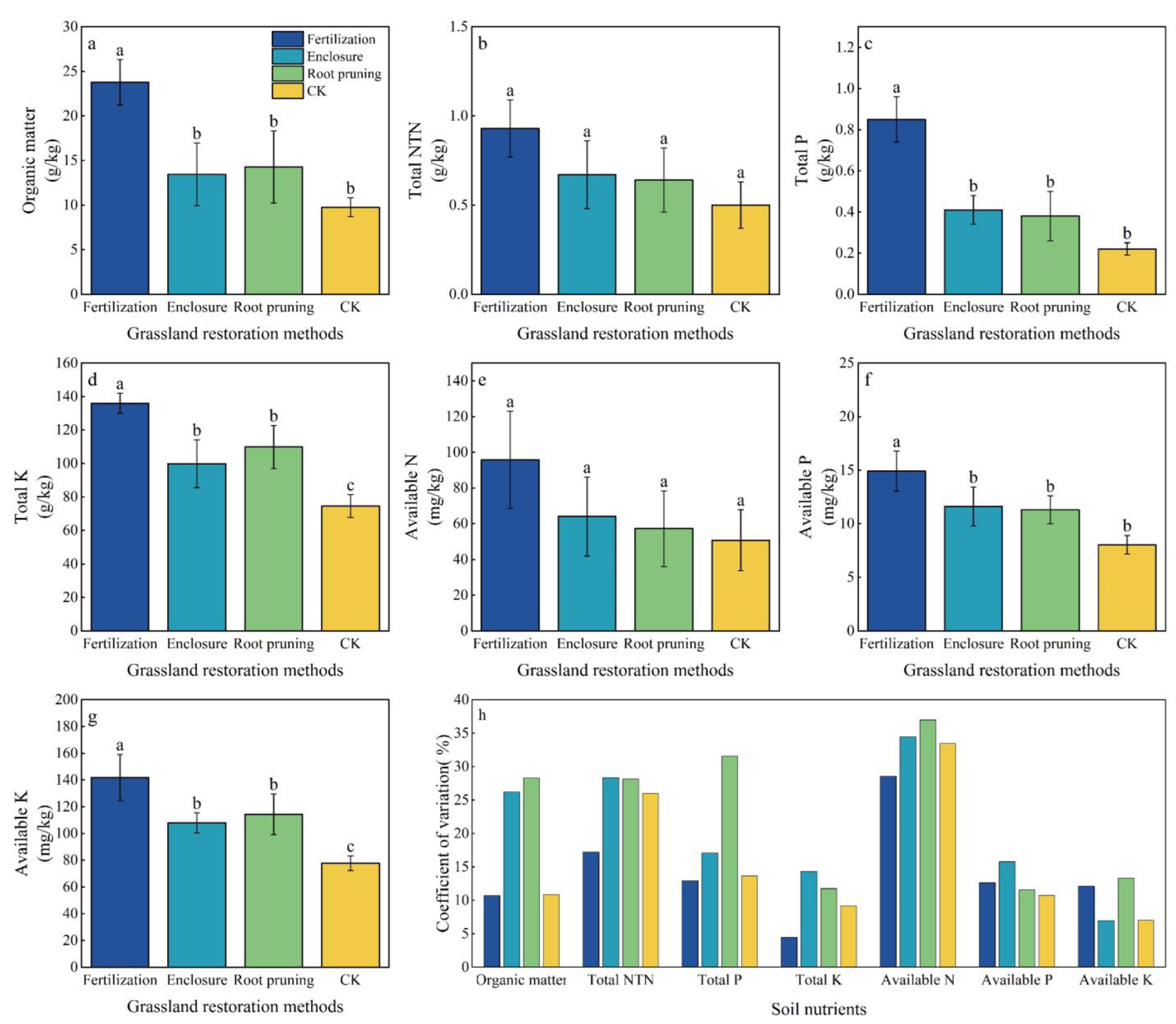The image showcases a series of detailed bar graphs arranged in a structured grid. The layout consists of three rows: the first and second rows each contain three bar graphs, while the third row contains two bar graphs. All the graphs share a common x-axis labeled "Grassland Restoration Methods," which include distinct categories—fertilization (navy color), enclosure (light blue), root pruning (green), and CK (yellow).

The top row of bar graphs illustrates various aspects of grassland restoration. The y-axes of these graphs represent different scientific measurements, such as organic matter, total NTN, and total P. The second row continues to depict grassland restoration methods with the y-axes detailing total K, available N, and available P. The bar colors are consistent with the legend found in the top left graph.

In the bottom row, the left bar graph still follows the grassland restoration methods with a y-axis representing available K. The graph on the far right is notably larger and shifts focus from grassland restoration to soil nutrients. Its y-axis covers various soil nutrient data points including organic matter, total NTN, total P, total K, available N, available P, and available K, with a particular emphasis on the coefficient of variation. The consistent use of color coding and labeling across the graphs provides a comprehensive comparison of different restoration techniques and their impacts on soil and plant metrics.